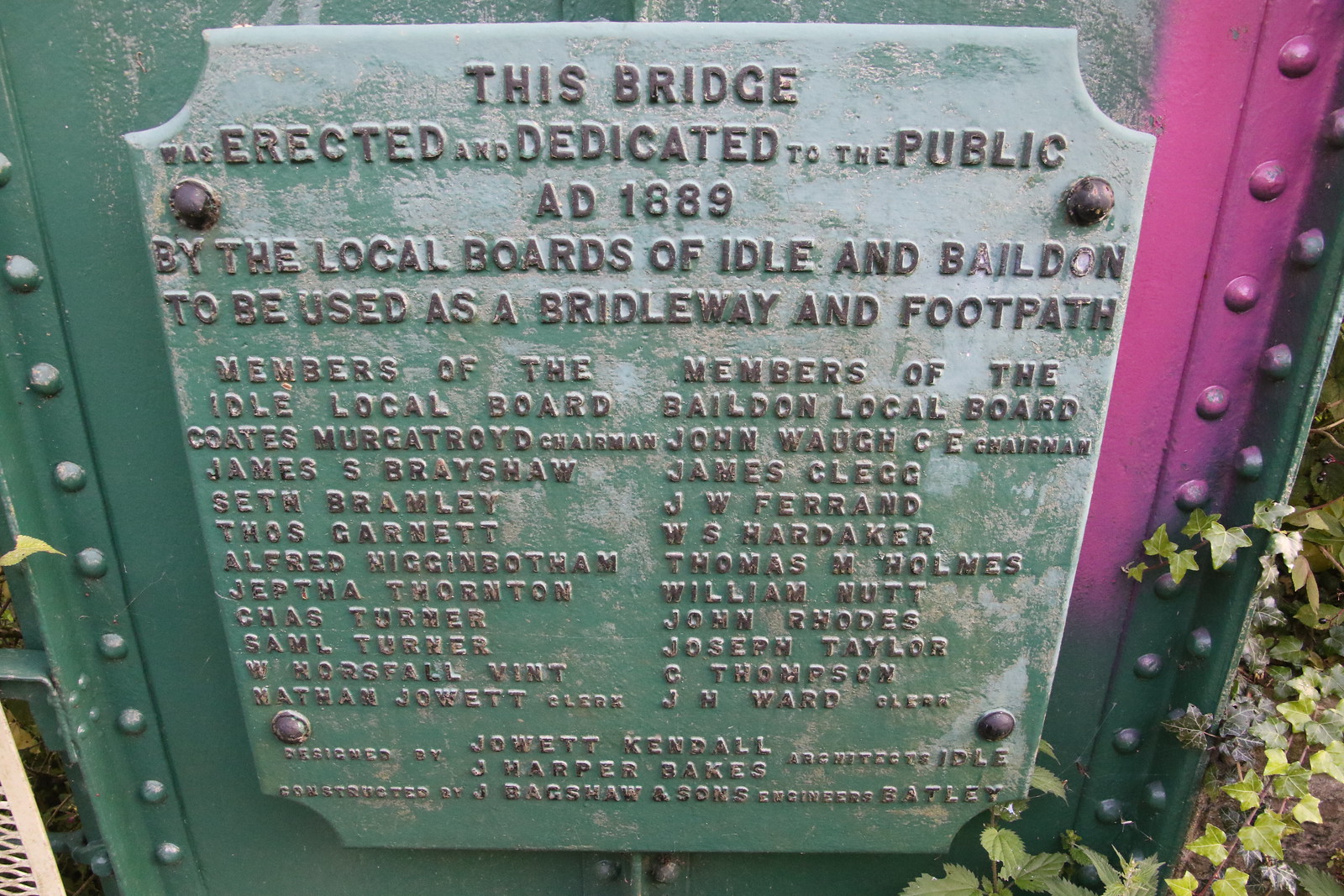The photograph, taken outdoors during the daytime, depicts a rectangular metal plaque attached to a green metal post, with a light green background and well-worn appearance. Measuring about six inches wide and four inches high, the plaque is firmly secured by four bolts, one at each corner, with small sections of the corners cut out. Despite some blurriness and glare, the raised brown lettering on the plaque reads: 

"This bridge was erected and dedicated to the public A.D. 1889 by the local boards of Idle and Baildon to be used as a bridleway and footpath. Members of the Idle Local Board: Coates Murgatroyd, Chairman; James S. Bradshaw; Seth Bramlett; Tom Garnett; Alfred Higginbottom; Jeptha Thornton; S. A. M. Turner; W. Horsfall; Vint Mattman; Jowett Kendall. Members of the Baildon Local Board: John Wallace, Chairman; James Clegg; J. F. Verand; W. S. Hardaker; Thomas Holmes; William Mutt; John Rhodes; Joseph Taylor; G. Thompson; J. H. Ward."

The plaque is also marked by signs of aging and has a purple spray paint stain to the right, near the rivets. The bottom of the plaque includes additional names but they are not clearly readable due to the wear and light reflection.